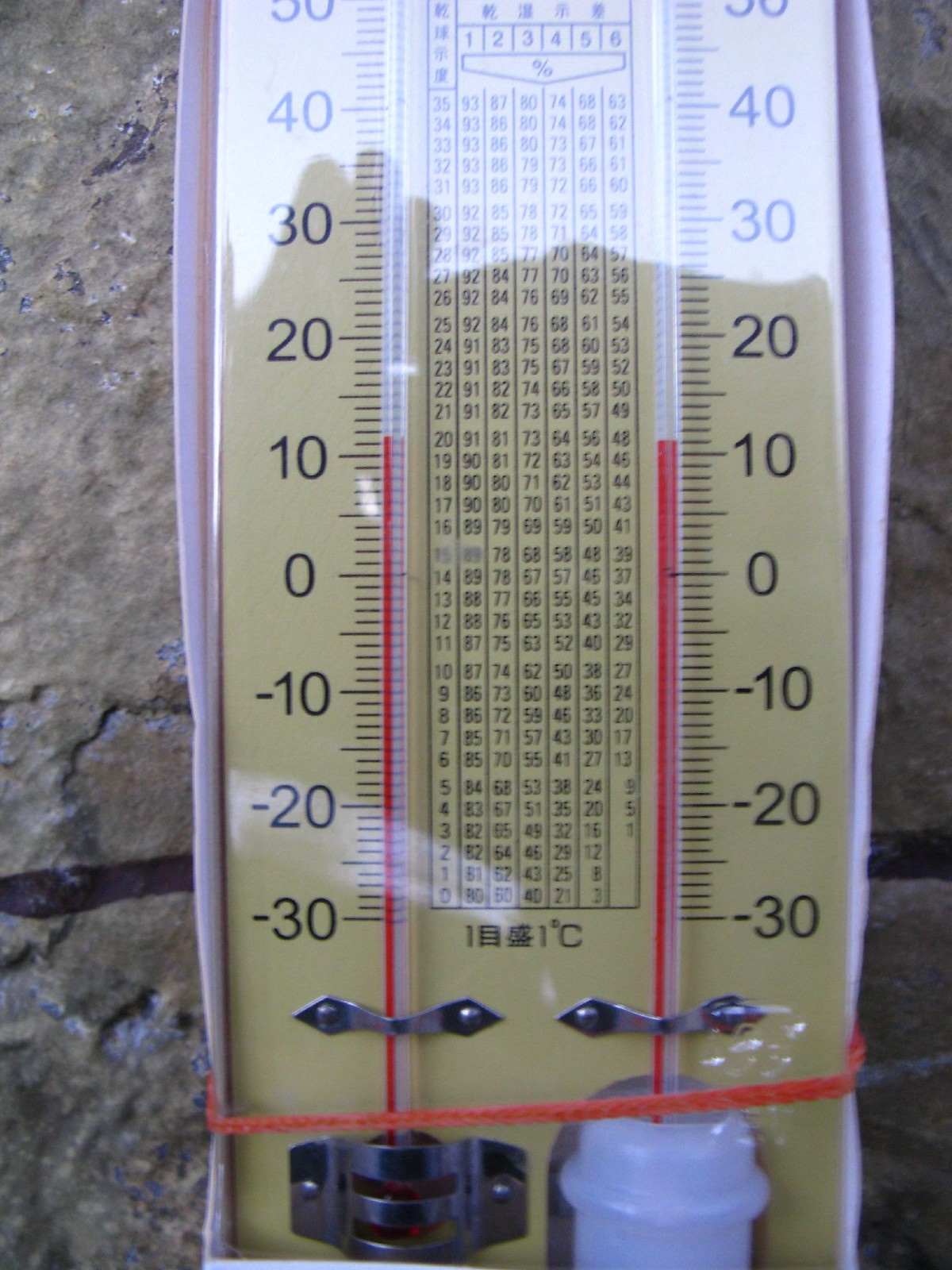The image features a dual thermometer setup placed on a wooden-colored, marble or stone background, suggesting it was taken outdoors. The composition includes two glass thermometers, each mounted on a distinct base. The thermometer on the left is secured by a metal base, while the one on the right is attached to a white base. Both thermometers display temperature readings ranging from -30 to 50 degrees, with an additional thermometer scale reaching up to 40 degrees and the partial reading of 50 degrees at the top.

Additionally, the image contains six columns marked with Asian characters, numbered from one to six, each followed by a percentage sign, indicating the presence of a hygrometer for humidity measurement.

Each thermometer is fastened to a white plastic case with metal clips. At the base of the plastic case, which appears slightly bowed on both sides, a red rubber band is visible near the metal clips. The plastic case features bright, reflected light at the top, which adds a striking element to the overall composition. Notably, both thermometers show a consistent temperature reading of 11 degrees. The entire setup appears meticulously designed and well-detailed.